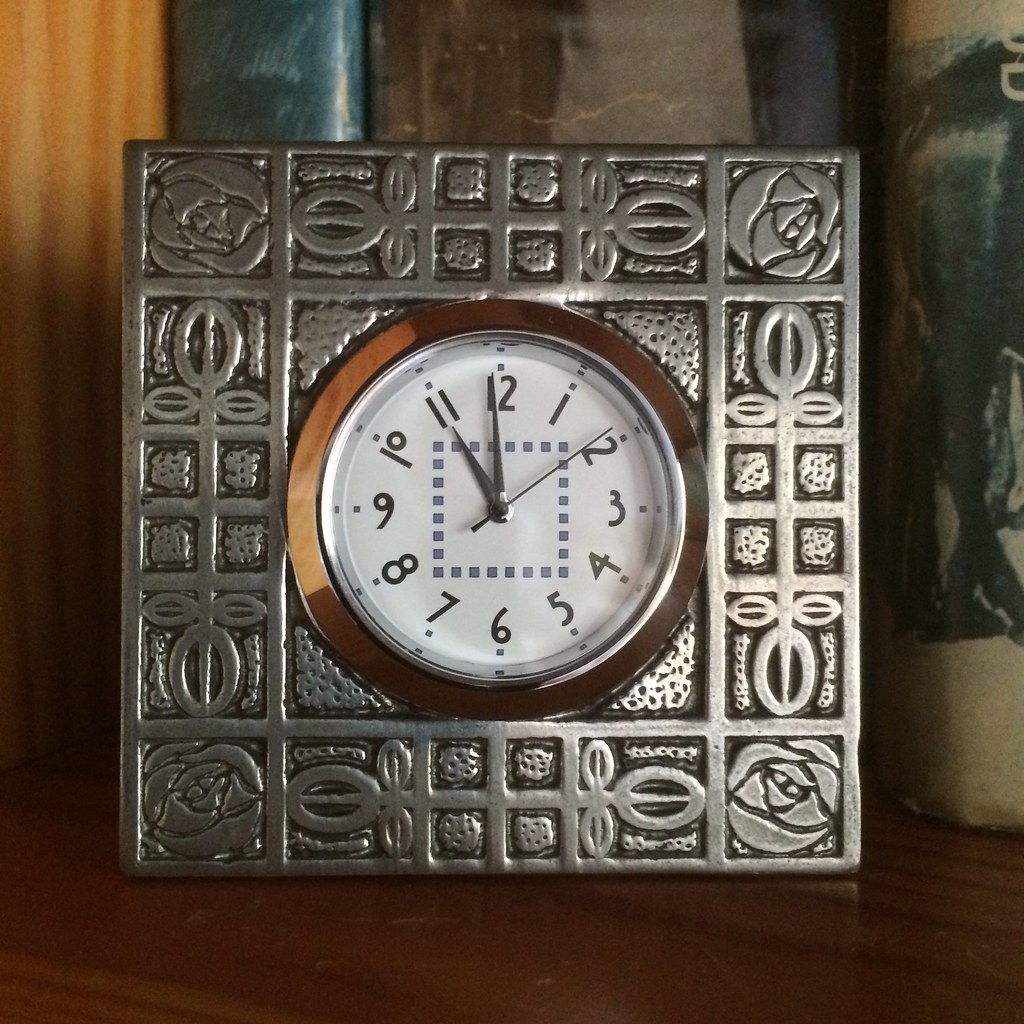This photograph captures an intricately designed analog clock resting on a wooden surface with a backdrop of books housed in a wooden shelf. The clock is encased in a square, ornate metal frame with a patterned border comprising squares, each adorned with detailed etchings—roses at the corners, interspersed with floral designs and a four-pane window motif. The clock itself is circular, set within a metallic housing, and features a white face with silver hands. A small mirrored border surrounds the clear glass cover, and the clock face displays an elegant font for the numbers. It is precisely 11 o’clock and 9 seconds, with the golden and silver hands pointing distinctively. This exquisite piece not only serves as a timekeeper but also as an artistic centerpiece, blending the charm of classic design with functional elegance.